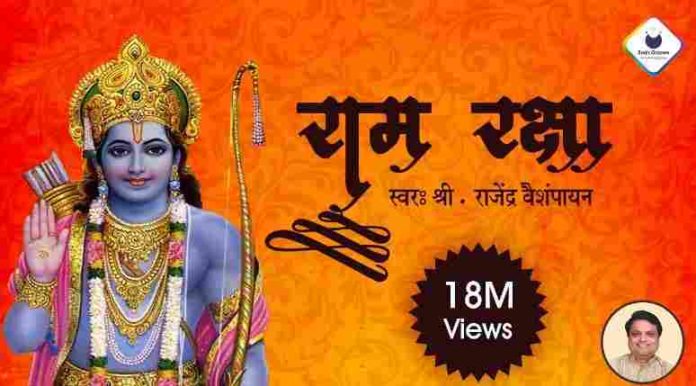The image features a vibrant gradient background that transitions from darker orange on the outer edges to a lighter orange at the center. Swirls of reds and grays add to the dynamic backdrop. Centralized slightly to the right is an artistic block of text in an elegant calligraphy-like script, possibly in a foreign language such as Chinese. Beneath this text, a seal resembling an award sticker displays "18M VIEWS" in white text, with "M" in uppercase and "views" in mixed case. Additionally, there's a small diamond shape with an illegible blue symbol inside. On the lower right corner of the image is a circular photo of a smiling man with brown hair slicked to the left, dressed in a white collared shirt. To the left of the image stands a striking blue-skinned figure adorned with a richly jeweled crown, ornate earrings, and multiple gold necklaces reminiscent of ancient Egyptian or Hindu attire. This figure, possibly a representation of Krishna, wields a golden bow in the left hand and has an arrow quiver on the back. The right hand is raised, either in a wave or a gesture to signal stop. The intricate details and cultural elements of the subjects, combined with the compelling use of colors and text, suggest it could be a poster or an ad.